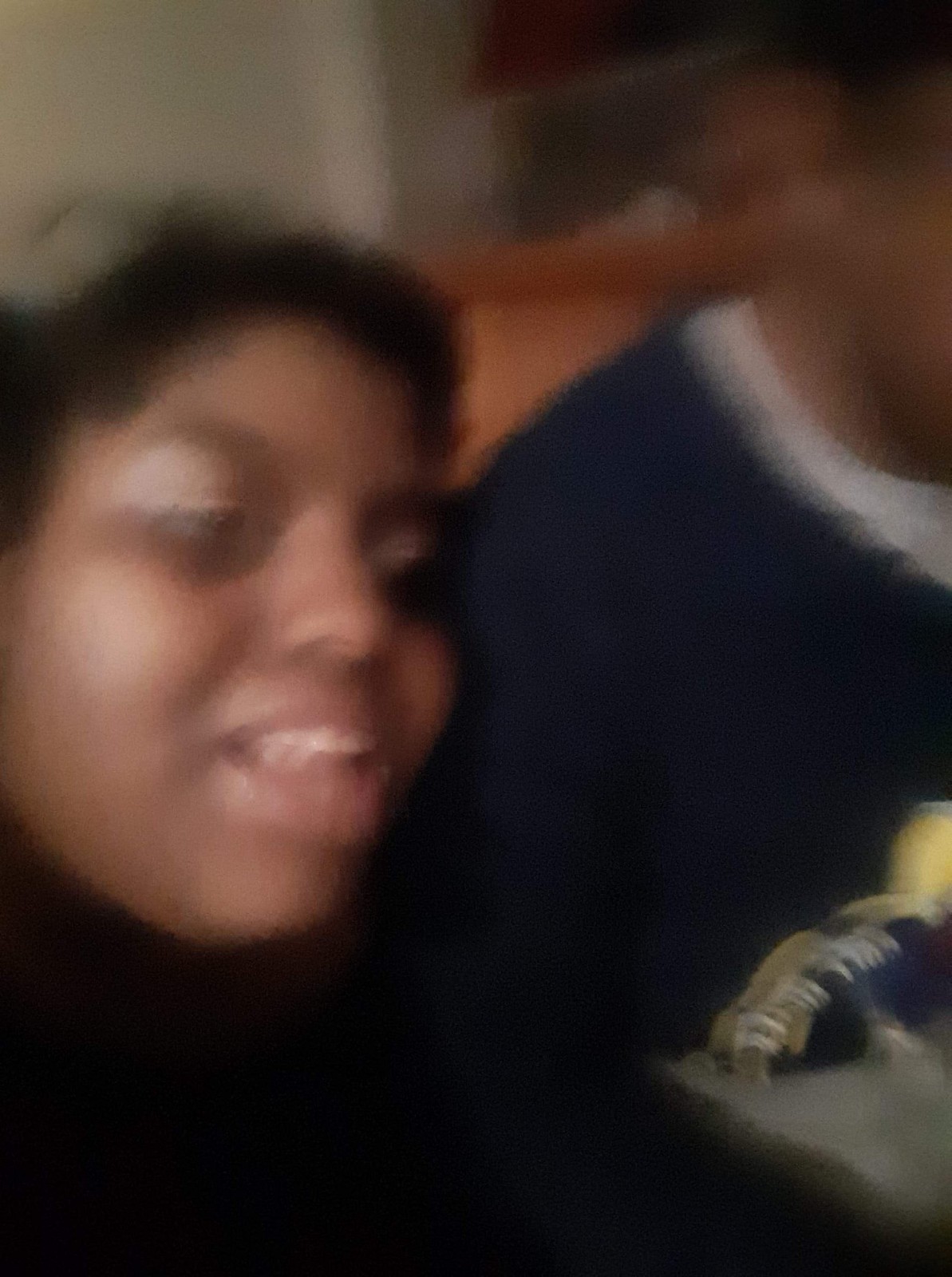In this very blurry photograph, a woman with brownish-black hair and possibly in her 20s or 30s is leaning against a man’s shoulder. Both appear to have brown skin. The woman, positioned on the left side of the image, has her mouth slightly open, with a hint of a smile, and is facing to the right. Her head tilts towards the man's shoulder, suggesting a close or intimate moment. The man is partially visible with an ear and part of his head shown in the top right corner of the image. He is wearing a blue sweater, which seems to have some print on the front, over a white shirt. Behind them, there might be a shelf or counter and a white wall. Additionally, there's an orange cabinet in the background. The photo is extremely blurry, making it challenging to discern further details, but in front of them is a blue, yellow, and white object that looks like items on a clothes rack.